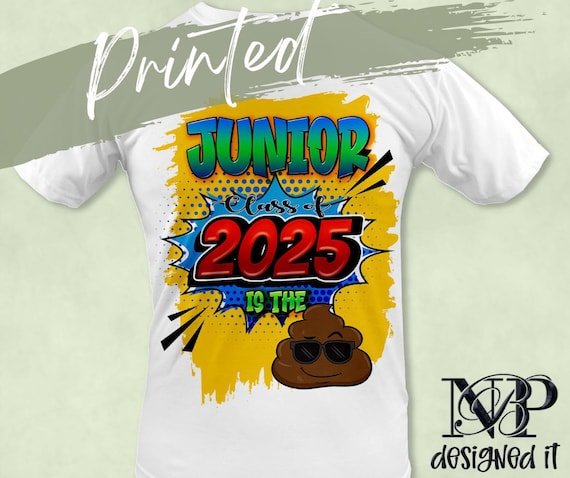The image features a white t-shirt adorned with an elaborate graphic design. At the center of the shirt is a prominent yellow splotch backdrop, over which the word "Junior" is displayed in a gradient that transitions from blue at the top to green in the middle, and back to blue at the bottom. Beneath this, a blue starburst pattern serves as the base for the black text "class of" which is followed by "2025" written in bold red. Completing the central design, the phrase "is the" appears in green, humorously followed by a brown poop emoji wearing sunglasses with a smile, indicating the phrase "Junior, class of 2025 is the shit."

Additionally, the shirt design includes the inscription "Printed" in white cursive at the very top left corner. On the bottom right, there is a distinctive logo that reads "NBP designed it," where the letters N and P are in block form and the ornate cursive B artistically wraps around both.